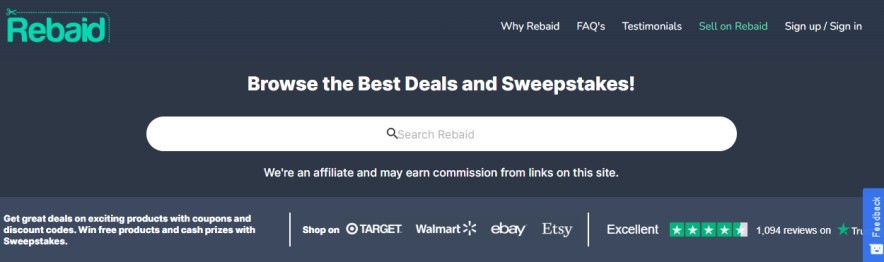The image showcases a webpage from a computer screen, prominently featuring the Rebate (Re-bade) website interface.

In the top left corner, there is a mint green label with the brand name “Re-bade.” Along the top right side of the interface, navigation options are displayed in white text: “Why Re-bade,” “FAQs,” “Testimonials,” “Sell on Re-bade,” “Sign Up,” and “Sign In.” The webpage is set against a sleek black background.

A highlighted text in the center reads, “Browse the Best Deals and Sweepstakes,” emphasizing Re-bade's main offering.

Below this, there is a large oval search box with the placeholder text “Search Re-bade,” intended for users to search the website's content.

It is noted that Re-bade operates as an affiliate and may earn commissions from links provided on the site.

At the bottom of the screen, a gray box contains promotional marketing text: “Get great deals on exciting products with coupons and discount codes. Win free products and cash prizes with sweepstakes,” encouraging user engagement.

In the middle of the page, there are icons of partnering retailers like Target, Walmart, eBay, and Etsy, offering users easy access to shop on these platforms via Re-bade. 

The website boasts a high user rating, displaying 4.5 stars out of 1,094 reviews on TrustPilot, rated as “Excellent.”